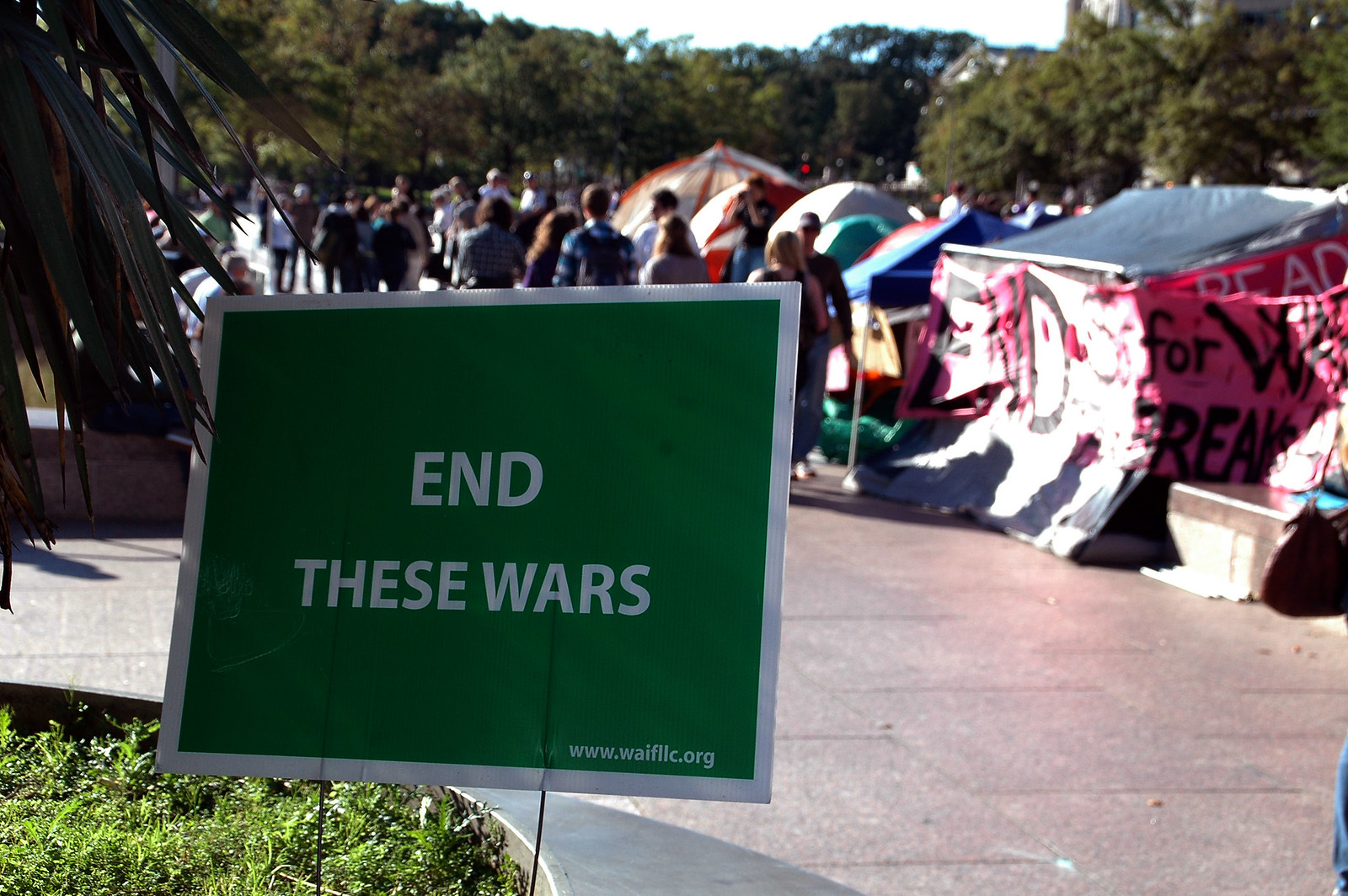The image captures a vibrant outdoor scene with a prominent green rectangular sign in the foreground. The sign features a white border and large white letters that read "END THESE WARS," with "www.waifllc.org" written at the bottom right. The sign is placed on a grassy area next to a tree. In the background, a large group of people faces away from the camera, walking along a sidewalk lined with numerous tents that bear various handwritten messages. The setting suggests a peaceful protest or a gathering advocating for the end of wars. The day is bright and sunny, with lush trees dotting the background, adding to the lively yet serene atmosphere of the event.